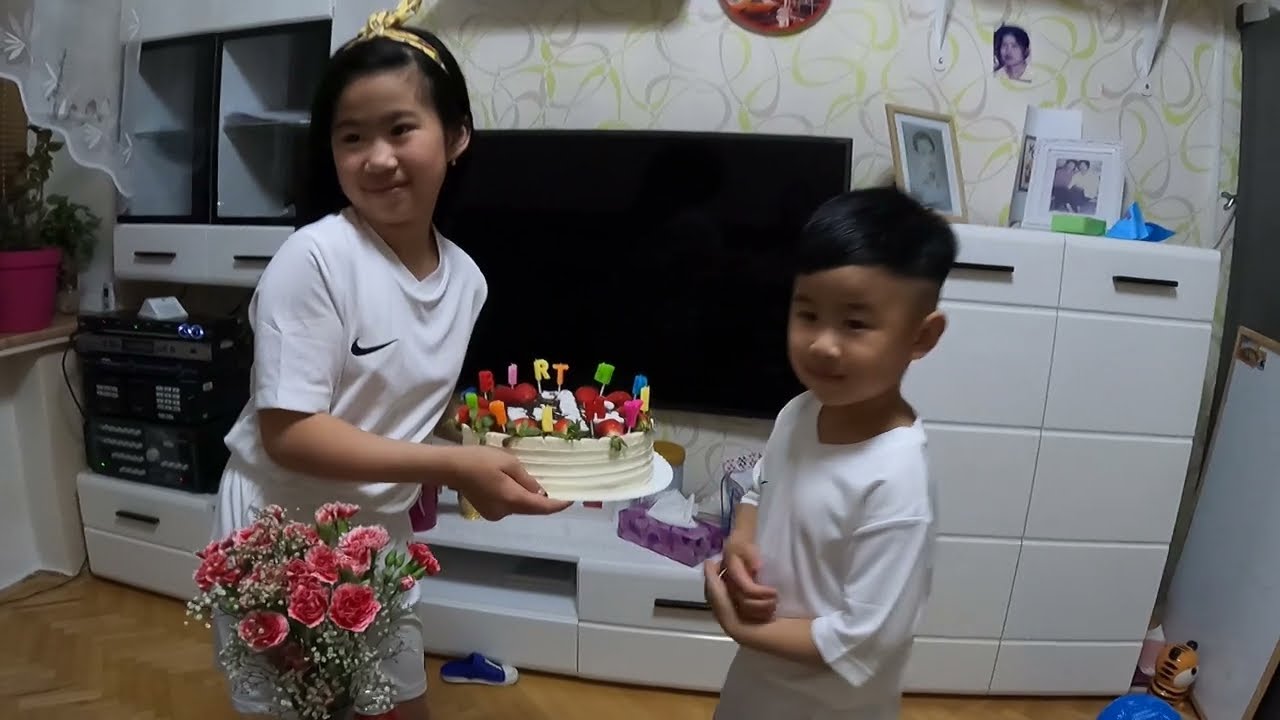The image depicts a warmly lit interior of a home, featuring two smiling Asian children, a girl on the left and a boy on the right. Central to the scene is a colorful birthday cake, decorated with multi-colored letters in shades of green, red, pink, yellow, orange, and blue, which the girl holds. A bouquet of pink flowers sits on the table nearby, adding a touch of festivity. In the background, white furniture can be seen along with a wall-mounted TV and a stereo system to the left. The children, both looking to the left, are the primary focus, radiating joy in this celebration captured within a comfortable, well-lit setting.